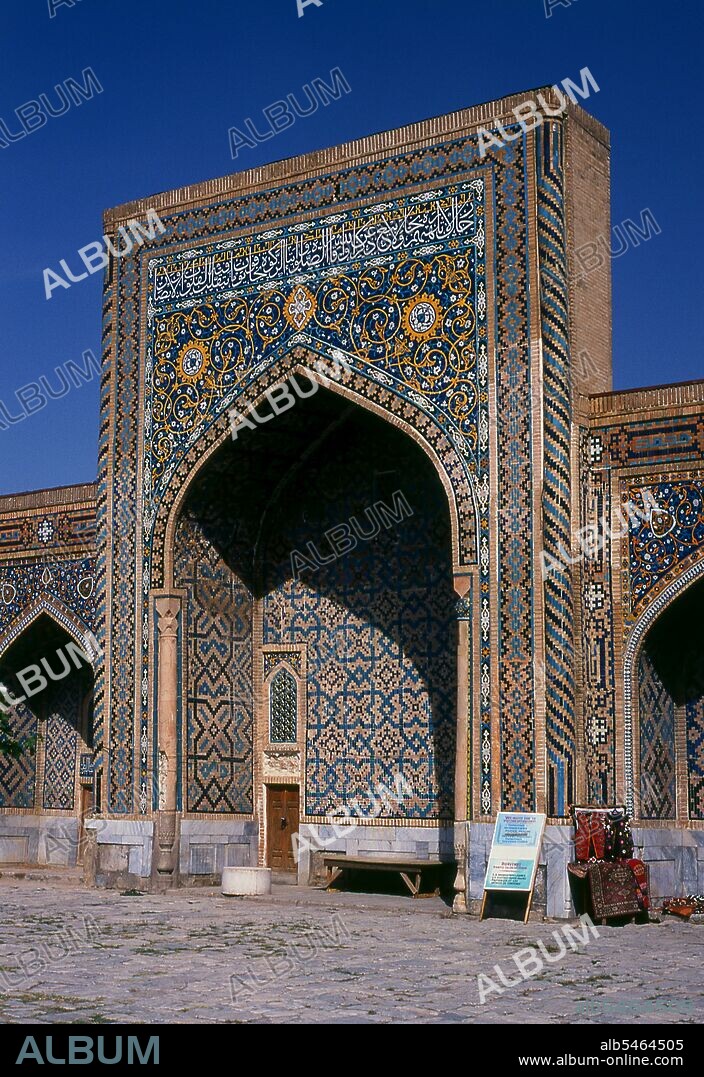This photograph captures a side-angled view of a highly detailed, ornate building that appears to be influenced by Moroccan or Indian architectural styles. The exterior is entirely adorned with exquisite, colorful tiles that exhibit intricate patterns resembling those found on oriental rugs, predominantly featuring shades of blue, white, orange, and gold. Central to the structure is a prominent pointed archway leading into a small hallway with a door, set within a rectangular façade complemented by additional smaller arched structures on either side. The vibrant backdrop of a clear blue sky enhances the photograph's vividness, emphasizing the building's grand scale as evidenced by the relatively smaller door at the base. The image is marked with multiple instances of the word "album" in a white or translucent font at a 45-degree angle, and a black border at the bottom inscribed with "www.album-online.com."